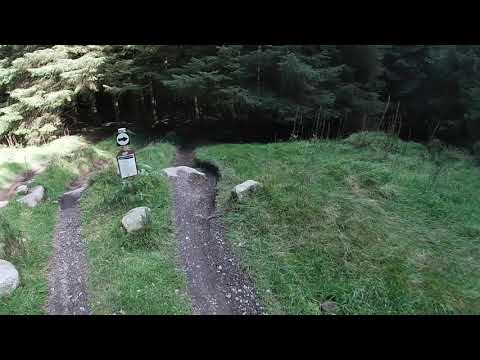The aerial image captures a scene of a dense forest with a clearing in front, showcasing an overgrown, long, matted grassy field. In the field, there are two distinct gravel paths characterized by their stony appearance; both paths appear to have been worn or carved out, with visible soil and submerged rocks. These trails, littered with large stones, lead directly into the dense woodland. Positioned between the trails is a noticeable signpost. The signpost features two signs: a circular white sign with a black arrow pointing to the right, and beneath it, a rectangular sign that contains text too small to be legible. The image reveals bright sunlight illuminating the right side of the clearing, while the left side remains in shadow, adding a contrasting light effect to the scene.